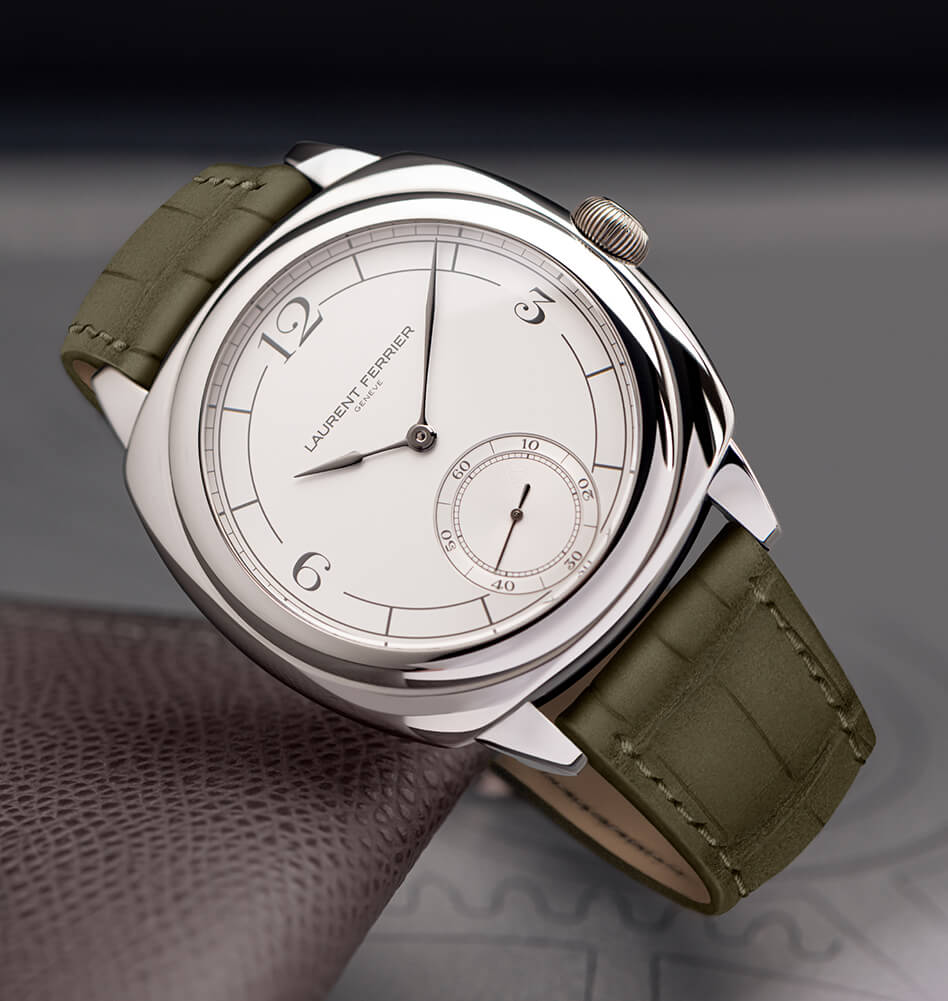This image features a close-up of a Laurent Ferrier wristwatch with a detailed brown alligator leather band meticulously stitched around the edges. The watch sports a silver or stainless steel case complemented by a crystal bezel. The classic white face is marked with prominent numerals at 12, 3, and 9 o'clock, while a sub-dial below the main face elegantly displays seconds, ranging from 10 to 60. The delicate timepiece shows the time as 10:09, with dark hands distinguishing the hours and minutes, and a single black hand for the seconds.

The watch is propped against a rich brown leather wallet, characterized by its worn, textured appearance. The setting is atop a surface adorned with impulsive gray scribbles and squiggly lines, blending into a background that transitions from black at the top to a blur of white.